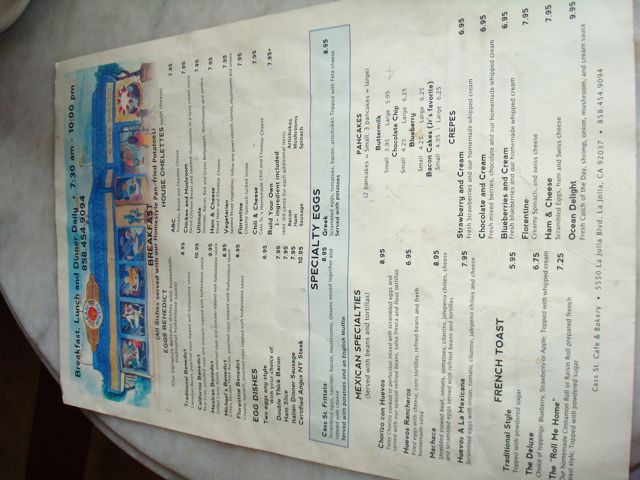This detailed photograph captures a restaurant menu, which is organized into four distinct quadrants, each elegantly bordered. The menu layout is traditional, with two sections on the left and two on the right. The light blue border accentuates the "Specialty Eggs" section. 

The top-left quadrant showcases various types of Eggs Benedict, including traditional, California, Mexican, Michael's, and Florentine. Each option, except for the California Benedict ($10.95), is priced at $8.95. The titles and descriptions are small, requiring a close look to read them. Both top quadrants are titled "Breakfast."

The bottom-left quadrant features "Mexican Specialties" and "French Toast," while the bottom right highlights a selection of crepes. The meticulous layout and detailed sections make it clear that this menu offers a variety of enticing breakfast options.